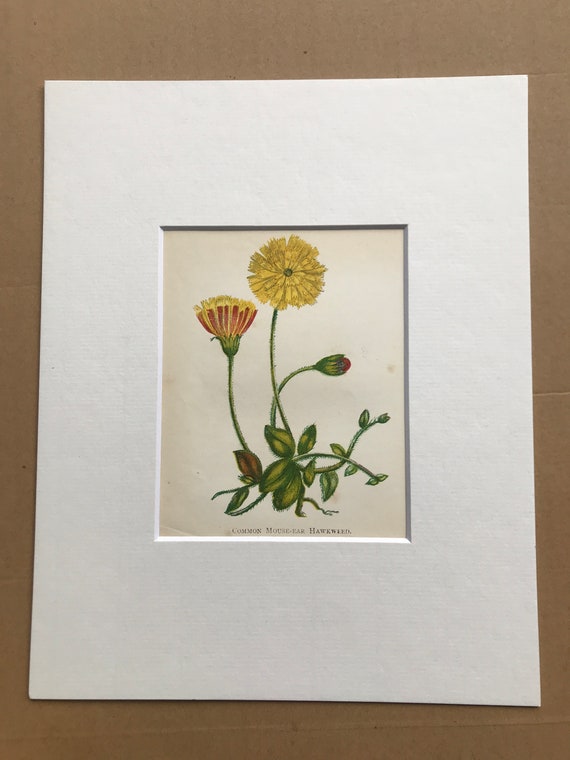The image depicts a framed illustration of flowers positioned against a medium brown background, which could be either a table or a wall. This vertically aligned rectangular picture features a large, thick white matte border surrounding the illustration. The artwork on off-white paper showcases three stems adorned with leaves and vines in varying shades of green with yellowish-green accents. 

On the left stem, a flower is in full bloom, facing the viewer, with a cluster of tiny yellow petals encircling a circular green center. Next to it, another flower, partially bloomed, reveals reddish petals still in a cone-shaped form. The third stem, slightly curved, bears a small bud with green petals partially encasing a rounded red tip. Below the illustration, three words are inscribed in black uppercase letters, of which "COMMON" is clearly legible, while the other words seem to be "MOUSE EAR" and "HAWKWEED," though they appear somewhat blurry. The illustration appears to potentially be a copy of an original color sketch and evokes a clinical, botanical style.